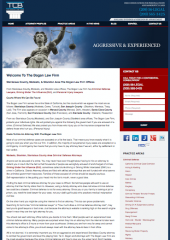The website features a very low-resolution design, with the acronym "TCB" in the upper left corner. To the right, under a dark blue band, is the contact information, followed by a black navigation band whose text is unreadable. 

Below this section, a full-width photograph depicts a statue of a woman holding scales, with some unreadable text in white on a blue background to the side. The photograph fades into a dark blue hue on the right side.

Under the photograph, there is a section filled with text in black and red that is illegible due to the poor resolution. To the far right, a vertically elongated rectangle contains four data fields, likely for user information such as name, address, email, and message.

Below this form are various social media icons, including recognizable Facebook and LinkedIn logos, along with other unreadable icons. Additionally, the right side contains a column of red, right-justified links against a gray background, matching the width of the aforementioned rectangle.